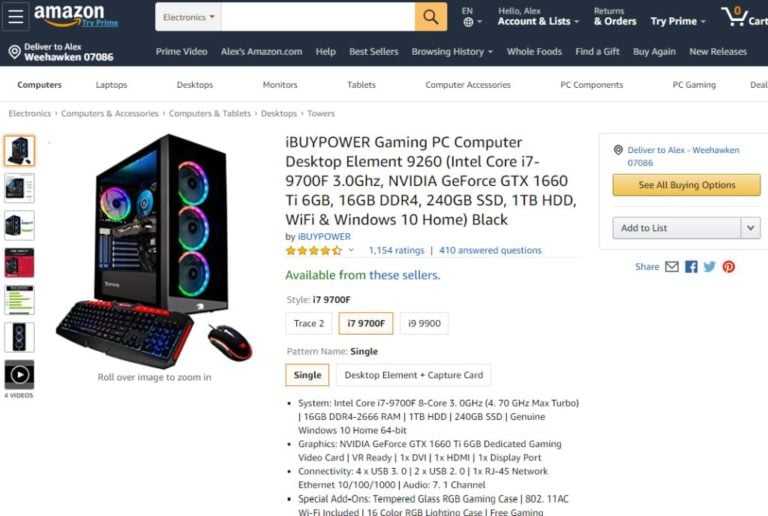This is a cropped screenshot of the Amazon.com website, focused on a product page featuring a desktop tower computer. The Amazon logo is prominently displayed in the top left corner of the banner, and the term "TriPrime" is visible in blue letters directly underneath it. To the right of the logo is a search bar, featuring a drop-down menu set to "Electronics."

Below the blue banner at the top, the page lists various shopping categories on a white background, spanning from the left edge to the right, though the right side of the page is cut off in the image. The first category listed is "Computers," which is highlighted in a darker font.

In the center of the page, there is a detailed description of an iBuyPower Gaming PC Desktop (Element 9260). The description is notably extensive. Below, it shows the product is by iBuyPower, includes star ratings, the total number of ratings, and the number of answered questions related to this computer.

On the left side of the page, there is a large, angled thumbnail image of the computer tower. Additionally, on the far left side, there is a vertical line of very small square thumbnails. The first thumbnail is highlighted with a red border and is identical to the large thumbnail image to its right.